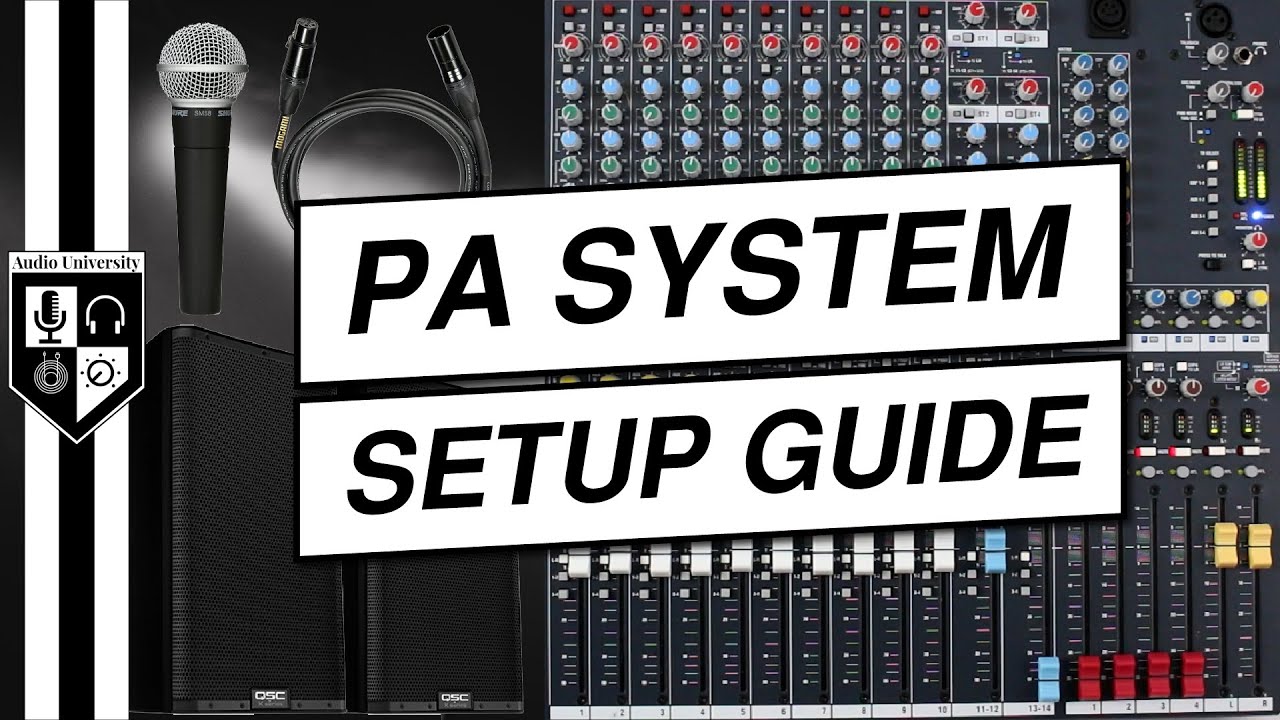This image appears to be the cover of a rectangular manual titled "PA System Setup Guide," prominently displayed across the middle. The layout is more extended horizontally than vertically. On the left side, there is a badge-shaped logo reading "Audio University," featuring icons of a microphone, headphones, a clock, and a volume knob within a shield. Surrounding this logo are alternating vertical stripes in black and white.

To the right of the logo, the image showcases various DJ and audio equipment. There are coiled coaxial cables, a handheld microphone, and a couple of speakers. Further right, an intricate control board is depicted, resembling equipment found in a music studio. This board is populated with numerous buttons, knobs, and sliders in vibrant colors including red, blue, light blue, green, white, orange, and yellow. The sliders are distinctive, with most being white, while a few are colored blue, red, and yellow. These sliders and buttons are scattered across different sections of the board, some intended for input and output controls, others for adjusting levels and sound quality, indicative of a comprehensive audio setup.